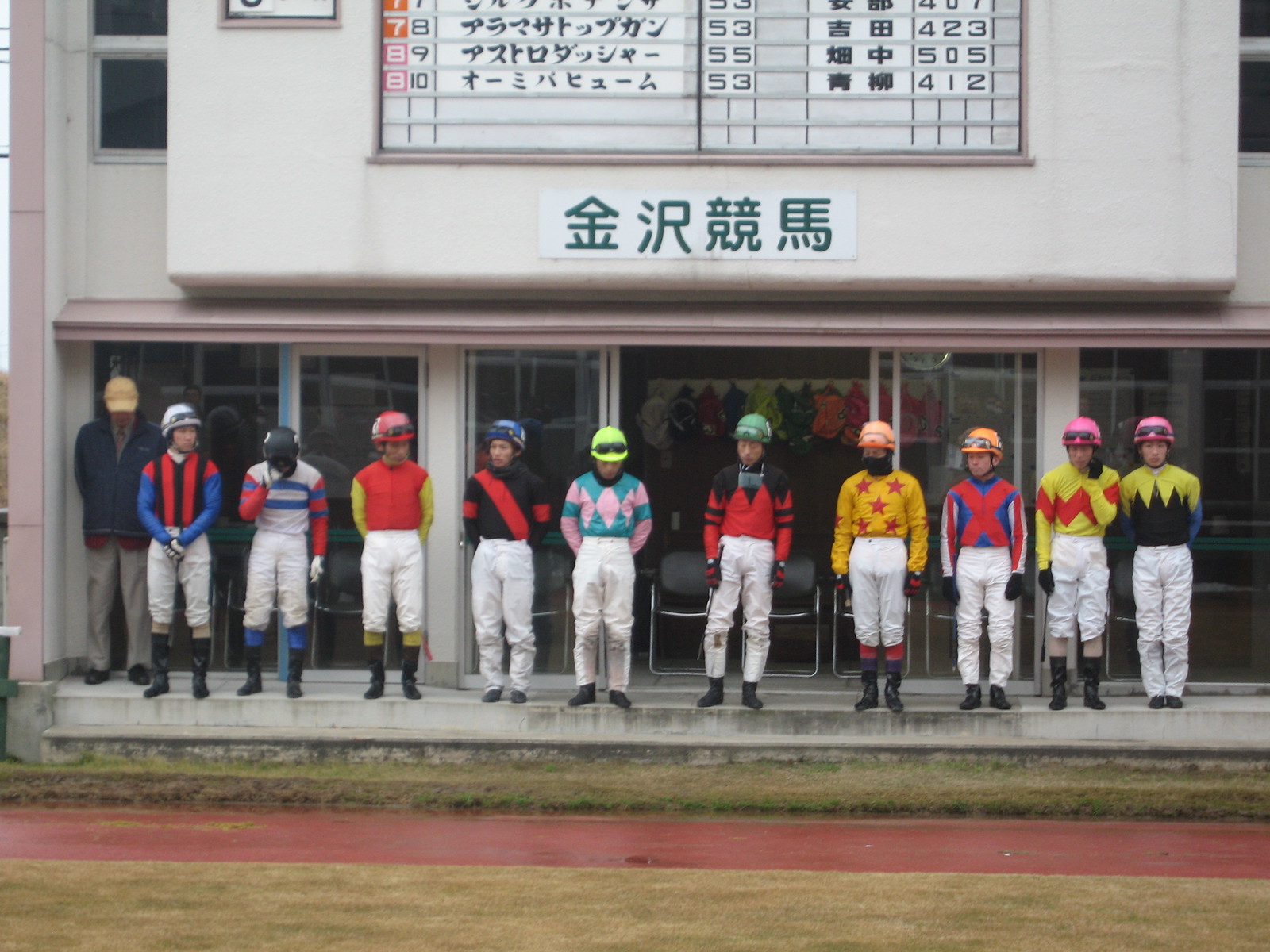The rectangular photograph captures an outdoor scene at a horse racetrack. In the background, there is a building with a glass front, featuring open doors and chairs neatly arranged. Behind the chairs, several vibrant jockey uniforms hang in a row on hooks. In front of the doorway, ten jockeys are positioned side by side, dressed in their distinctive attire of traditional white pants, black boots, colorful tops, and helmets. The uniform colors vary, including a yellow top with red stars, a black top with a red sash, a blue top with pink diamonds, among others, and the helmets match these color schemes with shades like pink, blue, yellow, red, black, and white. Above them, signage displays text in Chinese characters, indicating scores and positions, although the specifics cannot be read. In the immediate foreground, a patch of grass separates the jockeys from the reddish-brown racetrack, suggesting they might be either posed for a photograph or standing attentively for a ceremonial event like the national anthem, given their stoic and still demeanor.